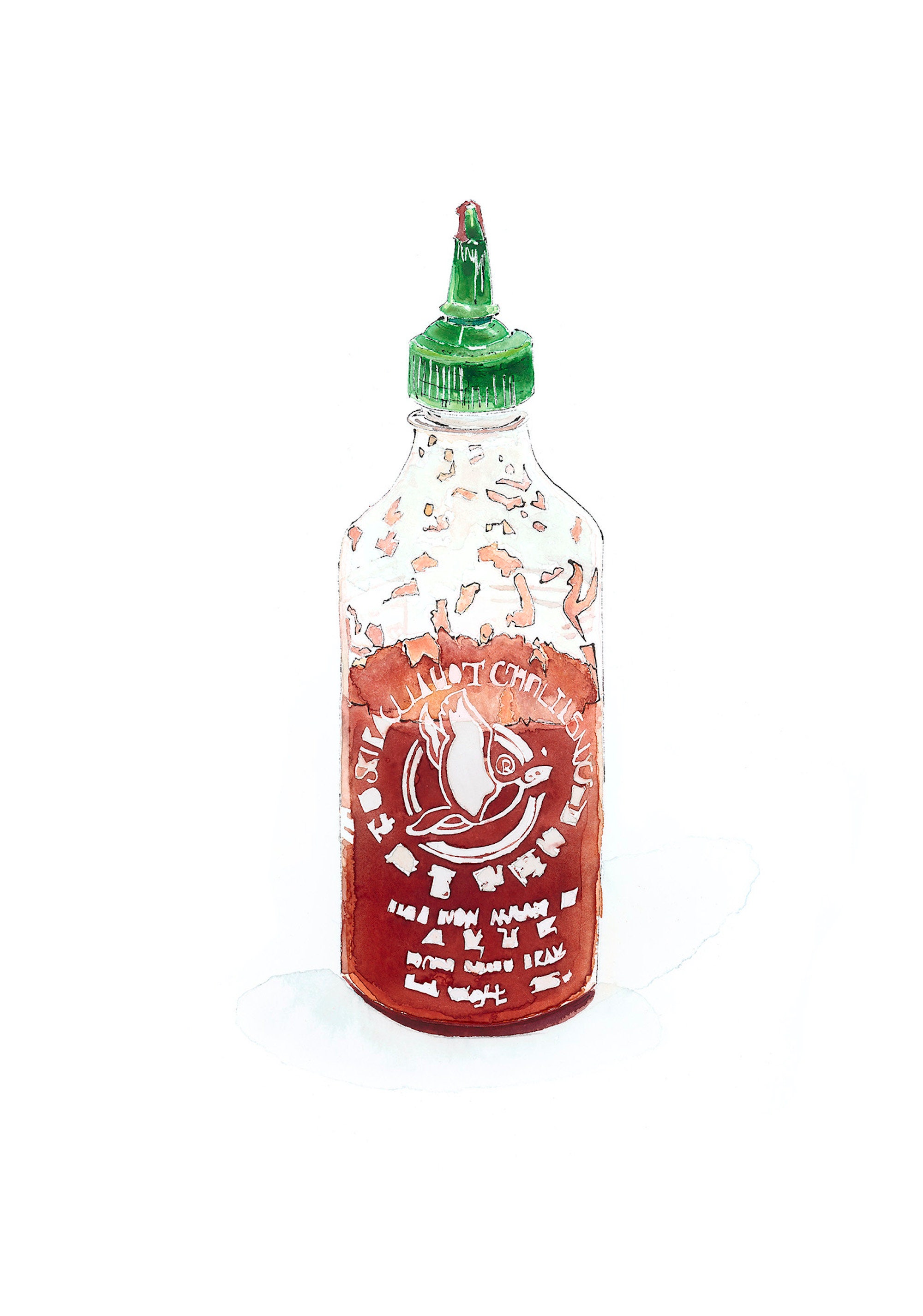The hand-drawn illustration depicts a clear squeeze bottle filled with a red to pinkish-brown liquid, reminiscent of ketchup or hot sauce, set against an entirely white background. The bottle features a distinctive green, ridged cap that tapers to a point. There's an image of a bird flying, encircled by a ring, on the front of the bottle, accompanied by illegible text arranged in a circular pattern around it and several white lines of text below. The surface of the bottle shows small droplets and smears of the red liquid inside, suggesting it was recently used or shaken. The detailed artistry of the label with its white images and inscriptions, along with the careful rendering of liquid inside, makes the bottle appear almost photorealistic.